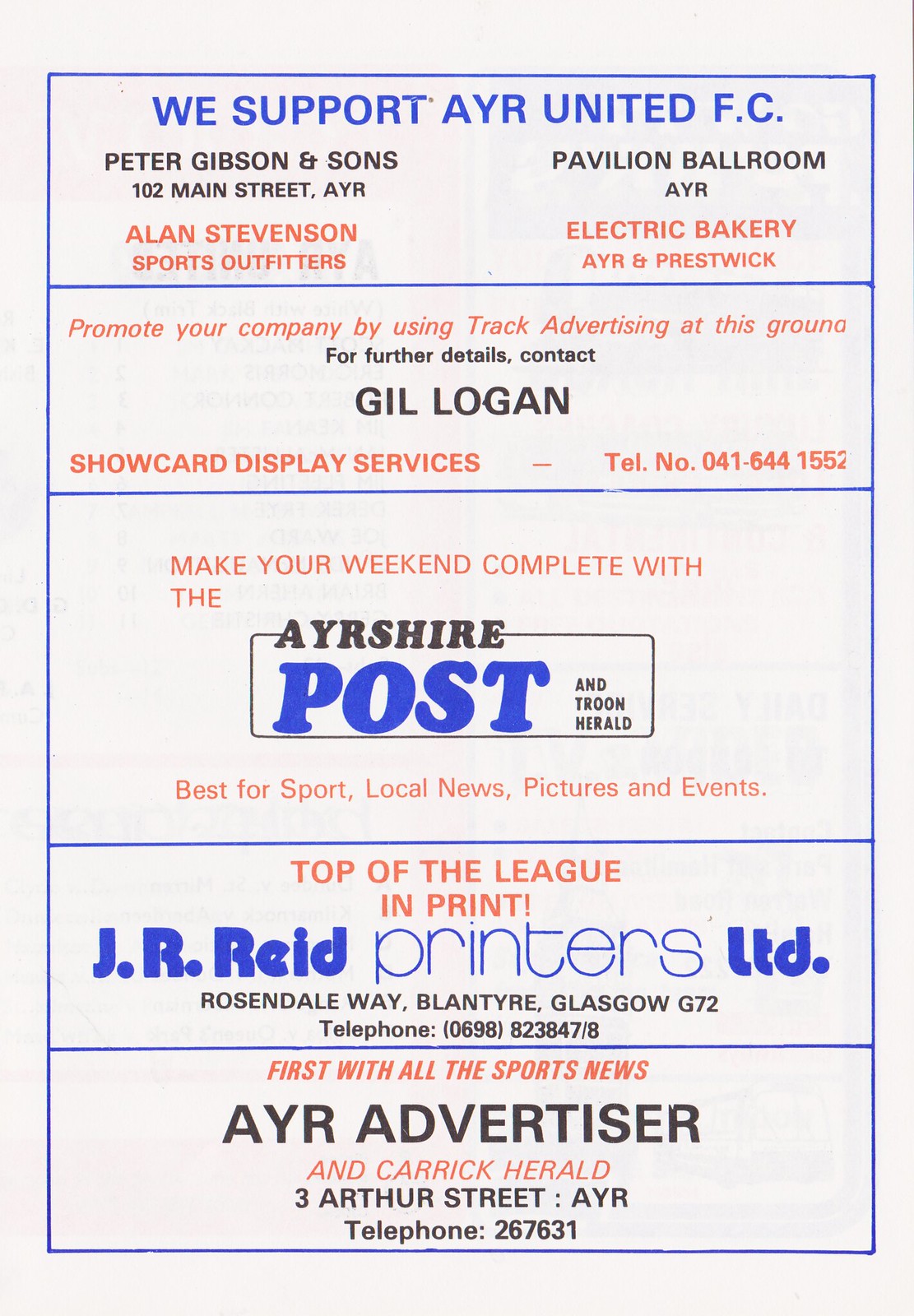This image, taken in portrait orientation, is a page from a printed sports program supporting AYR United FC. It features a light gray background with blue pinstriping dividing the page into five horizontal sections, each containing various advertisements from local sponsors. At the top, a blue headline reads, "We support AYR United FC." Below, the first section features sponsors: "Peter Gibson and Sons, 102 Main Street, AYR" and "Pavilion Ballroom, AYR" in black print, and "Allen-Stevenson Sports Outfitters" in red print, followed by "Electric Bakery, AYR, and Prestwick." The next box includes a red advertisement encouraging track advertising, with contact details for "Gil Logan" in black print, followed by "Show Card Display Services" in red print, and a telephone number.

The middle section promotes the "AYR Shire Post" with the text "Make Your Weekend Complete with The" in red, "AYR Shire" in black, "Post" in bold blue, and "and T. Roone Herald" in black, followed by "Best for Sport, Local News, Pictures, and Events" in red beneath it. The section second from the bottom features "Top of the League, In Print" in red, "J. R. R. Reed Printers, LTD." in blue, and "Rosendale Wave, Lantyre, Glasgow, G72" with a telephone number in black. The final section at the bottom highlights the "AYR Advertiser and Carrick Herald" with "First with All Sports News" in red, and address details in black print. The overall style of the publication is a traditional black-and-white print with spot colors of red and blue ink, creating a visually striking page dedicated to showcasing the sponsors and their support for the football team.